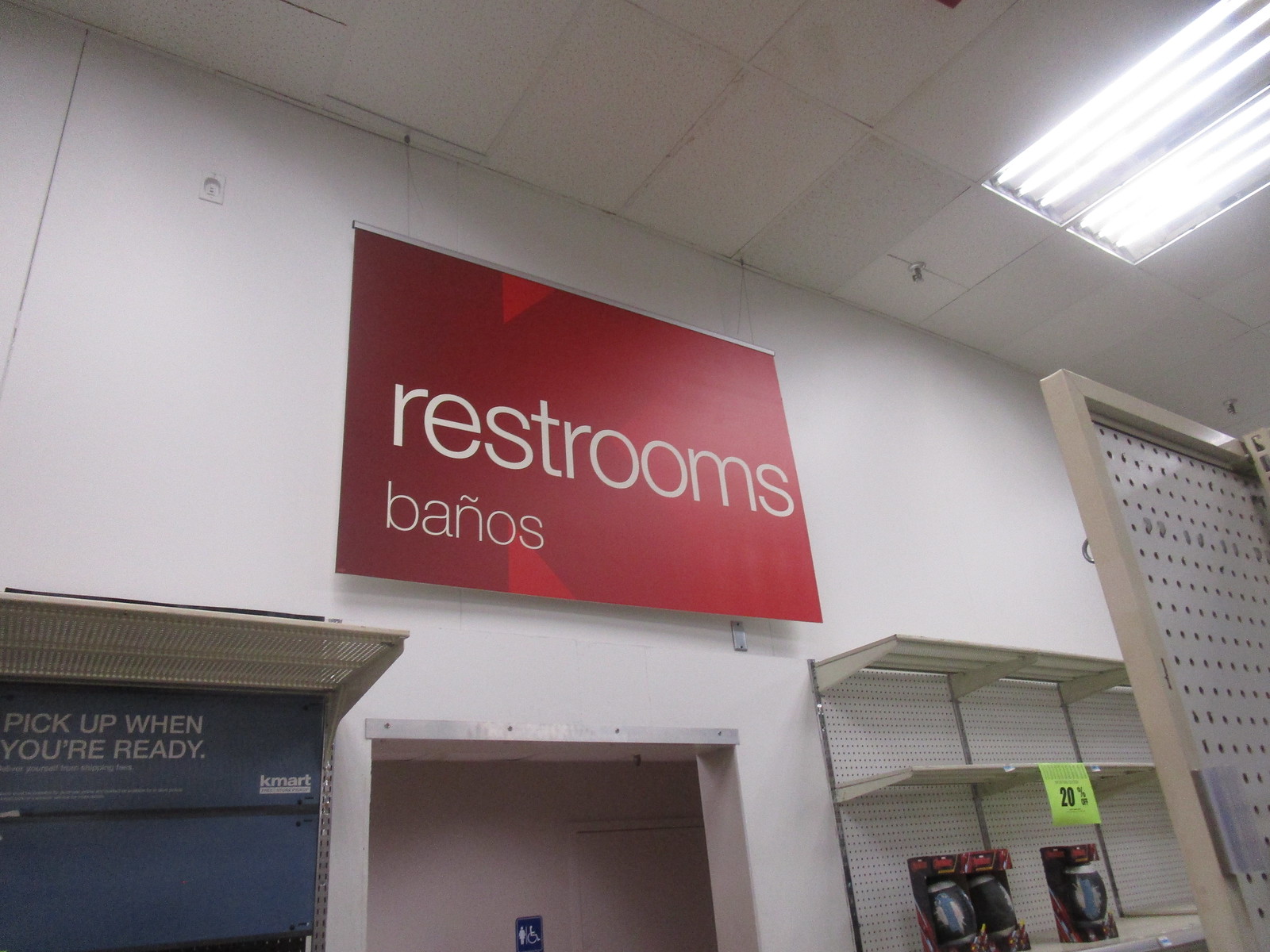This image portrays a section of a store with a modern, industrial design. The scene is dominated by light gray walls and a matching light gray ceiling, both adorned with prominent overhead lights and visible sprinkler systems. A window situated towards the back is fitted with black blinds and bears a sign that reads, "Pick up when you're ready." To the right, there are shelves: one shelf holds three footballs, while a larger beige-colored shelving unit features a perforated background. Also visible is a doorway marked by a large red sign that reads "Restrooms" in white text, with "Baños" indicated below.